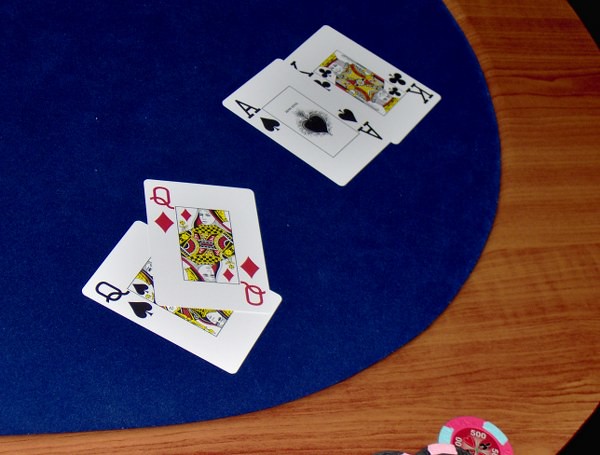The image captures a poker table with a dark blue felt surface, devoid of players or hands. Prominently displayed are four playing cards: the Queen of Diamonds laying diagonally across the Queen of Spades, and the Ace of Spades atop the King of Clubs. To the side, a hot pink poker chip adorned with green details and a clearly visible denomination rests alongside a light pink and black chip. The round table's edge is visible against a shadowy background that hints at a dark floor beneath. The scene is lit, yet the light source leaves no reflective glare on the table.